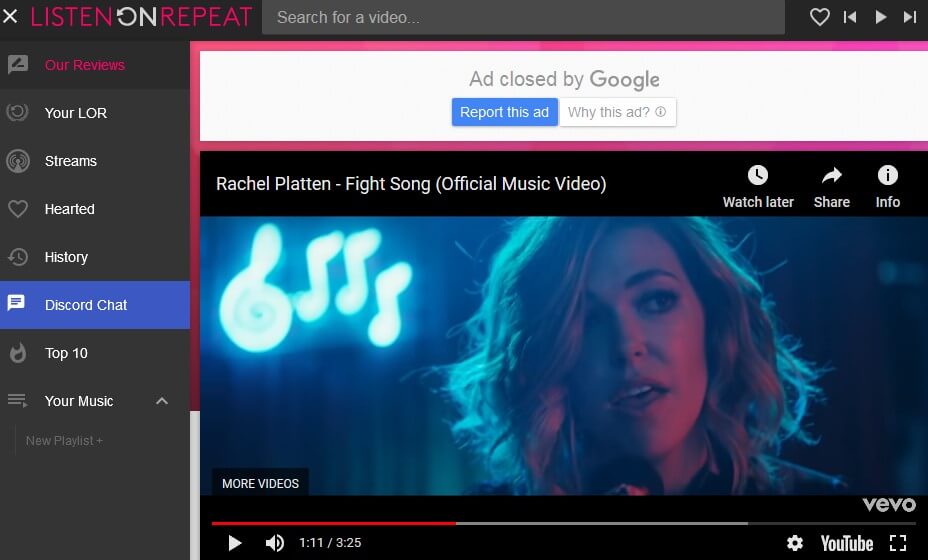ListenOnRepeat Website Interface with Rachel Platten's "Fight Song" Paused at 1:11

The website ListenOnRepeat features a sleek dark theme, creating a visually striking interface. At the upper left corner, a header bar stretches across the top, highlighted by a white "X" for closing. The title "LISTEN" in hot pink is prominently displayed, followed by "ON" in white with a replay arrow cleverly forming the "O," and "REPEAT" in hot pink to complete the branding. 

A gray search bar invites users to "search for a video..." in lighter gray text. To its right, icons for a white outlined heart, skip to the left, play, and skip to the right align neatly.

The left navigation bar, in darker gray, showcases a chat bubble with a pencil and paper icon, signifying "Our Reviews," which is currently highlighted. Beneath it, options labeled "Your L.O.R" with a replay arrow inside a fishbowl icon, "Streams" with a headset-like circle, "Hearted" represented by a gray heart outline with a black center, "History" with a standard history icon, "Discord Chats" with a blue background and white text, "Top Ten" featuring a flame icon, and "Your Music" with an upward arrow are visible. "New Playlist +" is shown in a darker gray with an icon resembling three horizontal bars and a play button.

Dominating the screen is Rachel Platten's "Fight Song" official music video from YouTube, paused at 1:11 out of 3:25. The video is two-thirds loaded with a red progress bar about one-third of the way. Watch Later, Share, and Info icons are at the top right of the video. 

The paused frame features Rachel Platten in a neon-lit bar scene, her hair partially covering one eye, and her mouth open as if singing. Behind her, a neon treble clef and three music notes glow in bright blue. 

At the top of the screen, a white ad bar by Google with options to "report this ad" in blue and "why this ad" with an info icon is visible. Additionally, the bottom right houses buttons for Settings, YouTube, and expanding the video to full screen, enhancing the interactive experience.